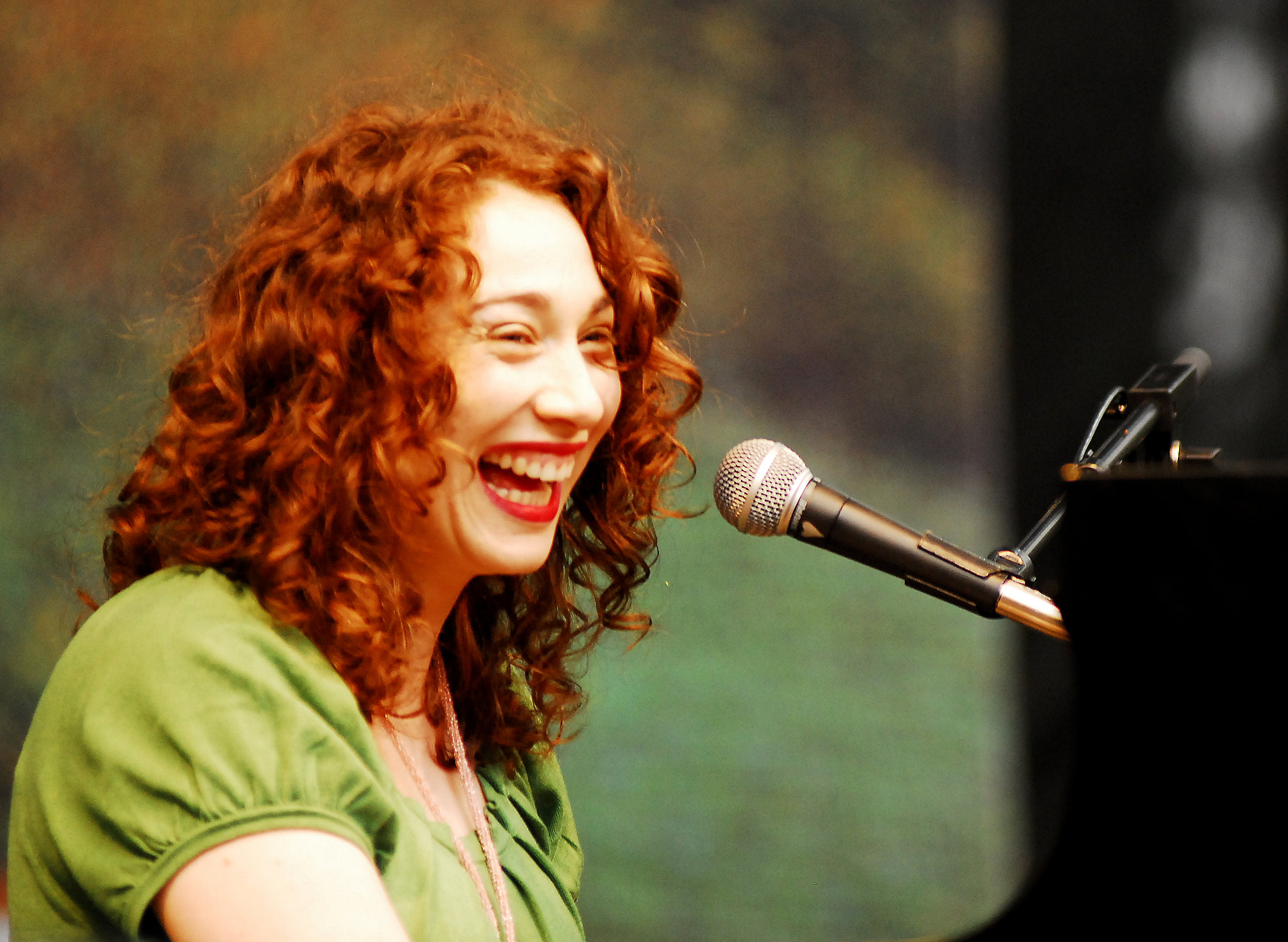The image captures a close-up of a woman with long, fiery red, almost orange, curly hair cascading past her shoulders. She is laughing heartily, evidenced by her wide-open mouth which reveals her teeth painted with red lipstick. Her fair skin is adorned with thin eyebrows, noticeable bags under her eyes, and pronounced dimples beside her nose. She is speaking into a black microphone, which is positioned to the right and mounted on a slender stand. The grip portion of the microphone is black, topped with a spherical mesh head. The microphone setup is possibly attached to a piano, suggested by visible components near the bottom right of the image.

The woman is dressed in a green short-sleeved top and accessorized with a pink bead necklace. Due to her laughter, her eyes are scrunched up, making their color indiscernible. The background is artistically blurred, transitioning from a green hue at the bottom to a brownish tone at the top, with a black section on the right side, further emphasizing her animated expression and colorful attire.